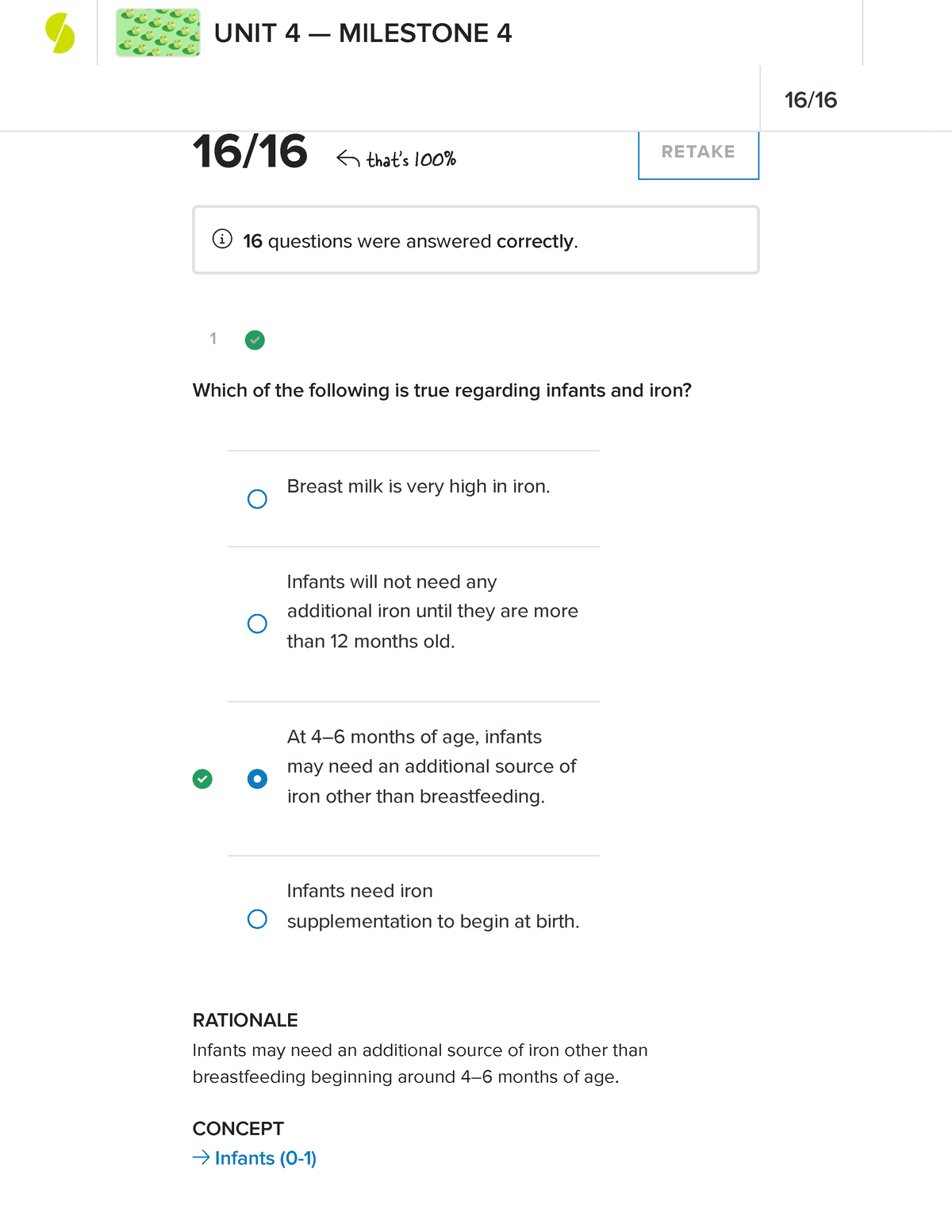The image appears to be a screenshot of a class-related webpage. It displays Unit 4, Milestone 4 with a perfect score of 16 out of 16, indicating that all 16 questions were answered correctly. One of the questions displayed reads: "Which of the following is true regarding infants and iron?" The answer options are: 
1. The breast milk is very high in iron. 
2. Infants will not need any additional iron until they're 1-12 months. 
3. At 4-6 months of age, infants may need an additional source of iron other than breastfeeding. 
4. Infants need iron supplementation to begin at birth. 

The third answer is marked as correct: "At 4-6 months of age, infants may need an additional source of iron other than breastfeeding." Below the question, a rationale explains that infants may need an additional iron source other than breastfeeding around 4-6 months. A provided link offers more information on this concept. 

The webpage suggests that the quiz is intended for learning purposes, perhaps by prospective parents, and allows retakes. It implies that the score does not affect any official academic record. A logo at the top left features a design resembling two offset halves of a circle, creating an 'S' shape.